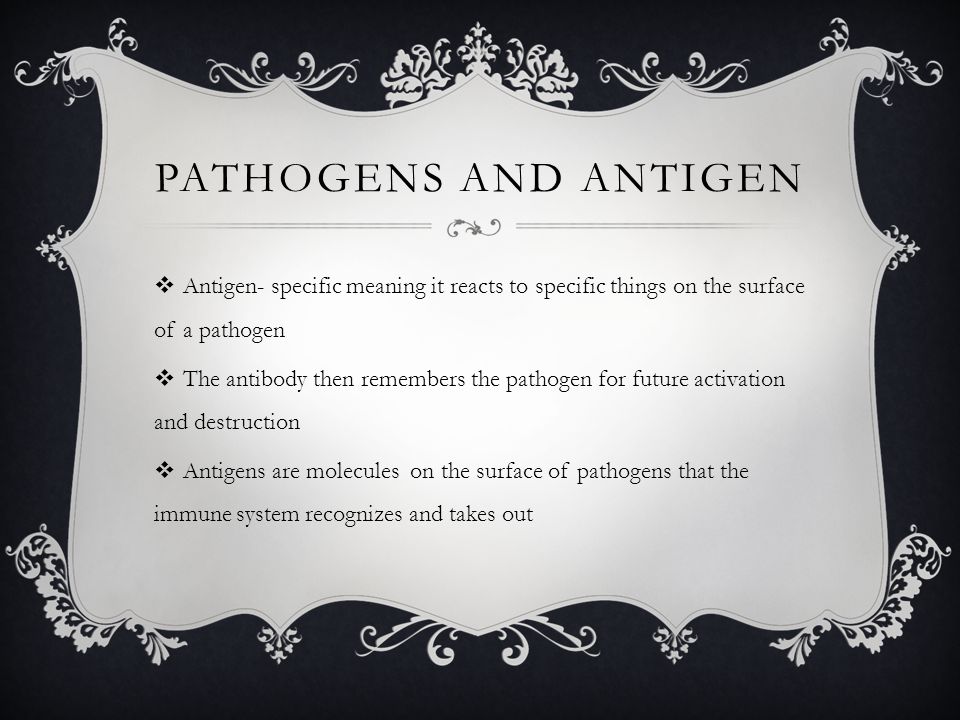The image features an elegant, textbook-like page with a white background set against a black backdrop, adorned with intricate, lacy, and leafy designs around its edges, reminiscent of a wedding announcement. At the top, the title "Pathogens and Antigen" is prominently displayed in black text, underlined by a decorative, sideways 'S' embellished with leaves. Below the title, three bullet points, marked by small diamonds, provide detailed information: 

1. "Antigen-specific, meaning it reacts to specific things on the surface of the pathogen."
2. "The antibody then remembers the pathogen for future activation and destruction."
3. "Antigens are molecules on the surface of pathogens that the immune system recognizes and takes out."

The central focus of the image is this detailed and stylish explanation of the relationship between pathogens and antigens, presented in a sophisticated format.